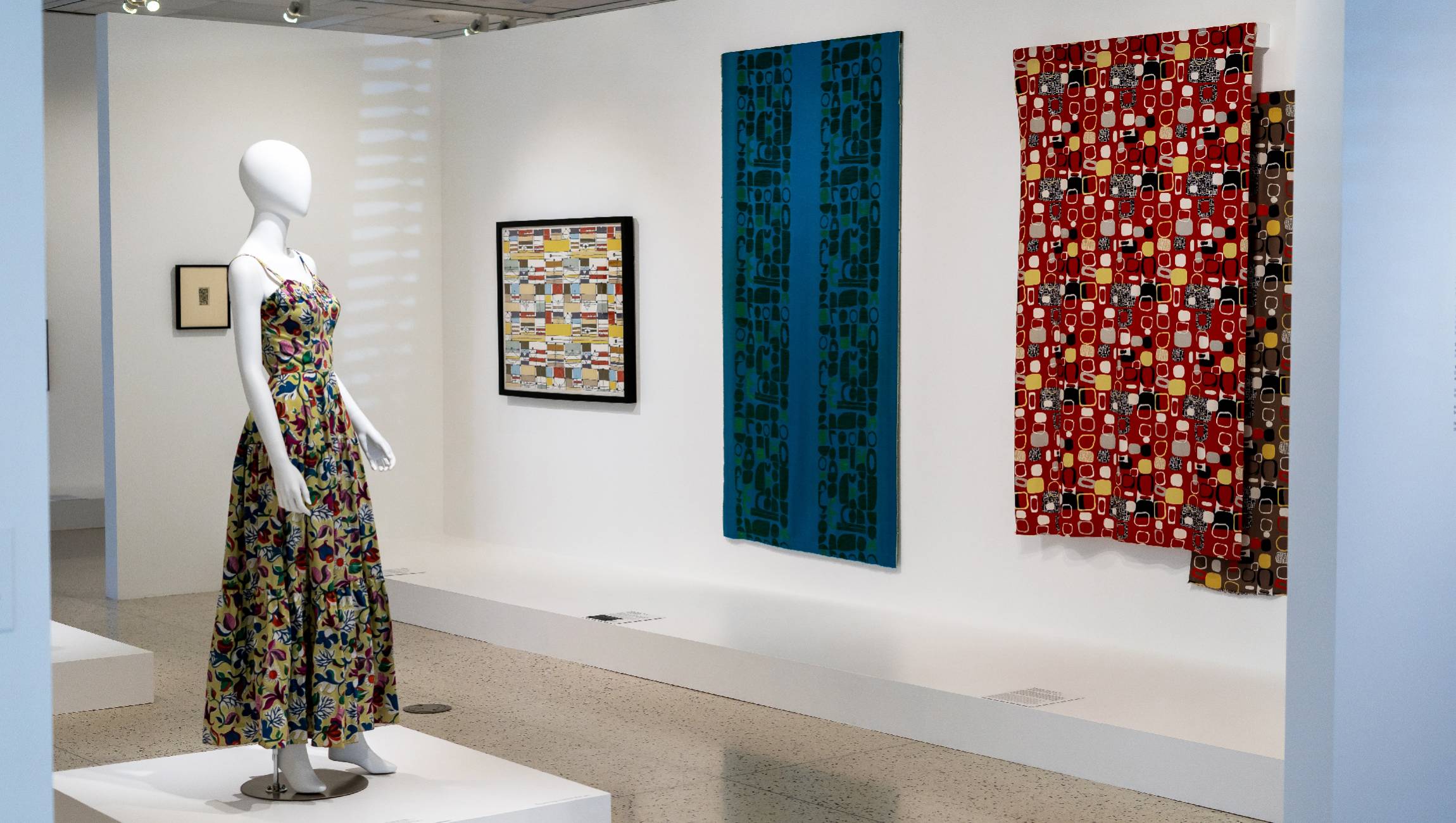In the photograph, the setting appears to be a gallery or museum, characterized by its white walls and tan tile flooring. Central to the image is an elevated platform featuring a white mannequin adorned in a dress with an artistic, hand-painted floral design, incorporating blue flowers, green foliage, berries, and a yellow background. The mannequin faces to the right. Behind it, the gallery walls display a series of modern art pieces and textile works. Noteworthy among these are a tan fabric with a black square and an inner gray rectangle, a multicolored quilt-like piece framed in black, a vertical blue tapestry with dark and light blue segments and black boxes, and another rectangular red tapestry embedded with squares in white, beige, yellow, and black. The diverse art pieces, some akin to tapestries with geometric patterns, reinforce the thematic coherence of a textile artist's exhibit.